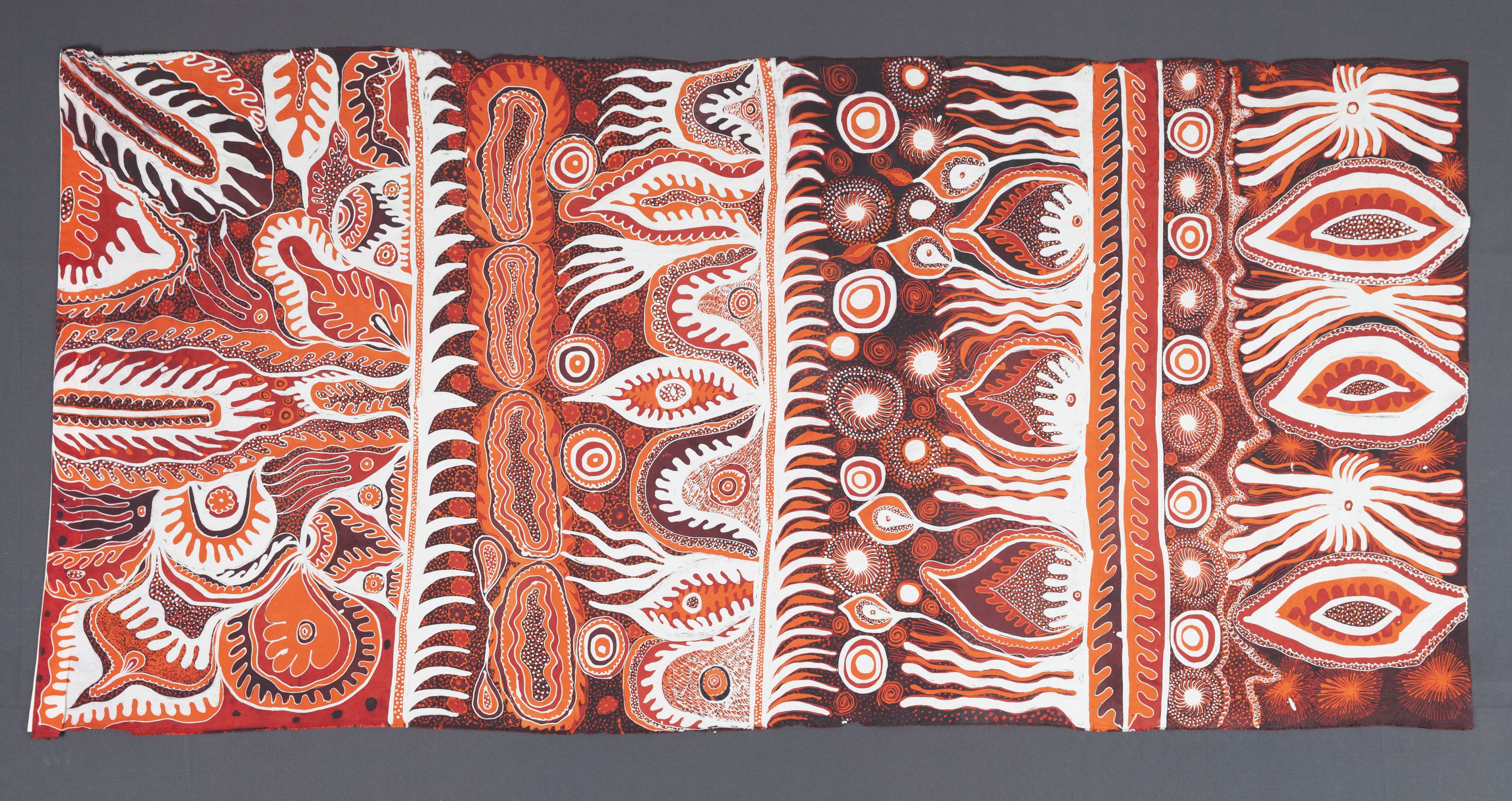The image depicts a detailed painting of a tribal rug or blanket with intricate designs, laid out against a gray border. The rectangular artwork is divided into four distinct sections, each featuring unique patterns and vibrant colors.

The first section on the left showcases a design reminiscent of bird feathers, incorporating a palette of dark gray, black, white, red, orange, and brown. This part features large, prominent feather or leaf shapes in various combinations of white, black, red, and white.

The second section is adorned with what appears to be different types of plant motifs, executed in complementary hues. The third portion is characterized by fiery patterns or abstract designs that might suggest a snake or dragon, utilizing shades of purple, orange, and red to create a dynamic visual effect.

The fourth and final section presents designs that evoke human eyes, rendered in red, white, and black. Additionally, this area includes elements that hint at African, Polynesian, or Aboriginal art styles, further enhancing the cultural richness of the painting.

The artwork contains no text or inscriptions, focusing solely on the visual impact of its lavish, multicultural designs. Overall, this striking painting captures a complex tapestry of symbols and colors, resembling a tribal blanket rich with historical and artistic significance.